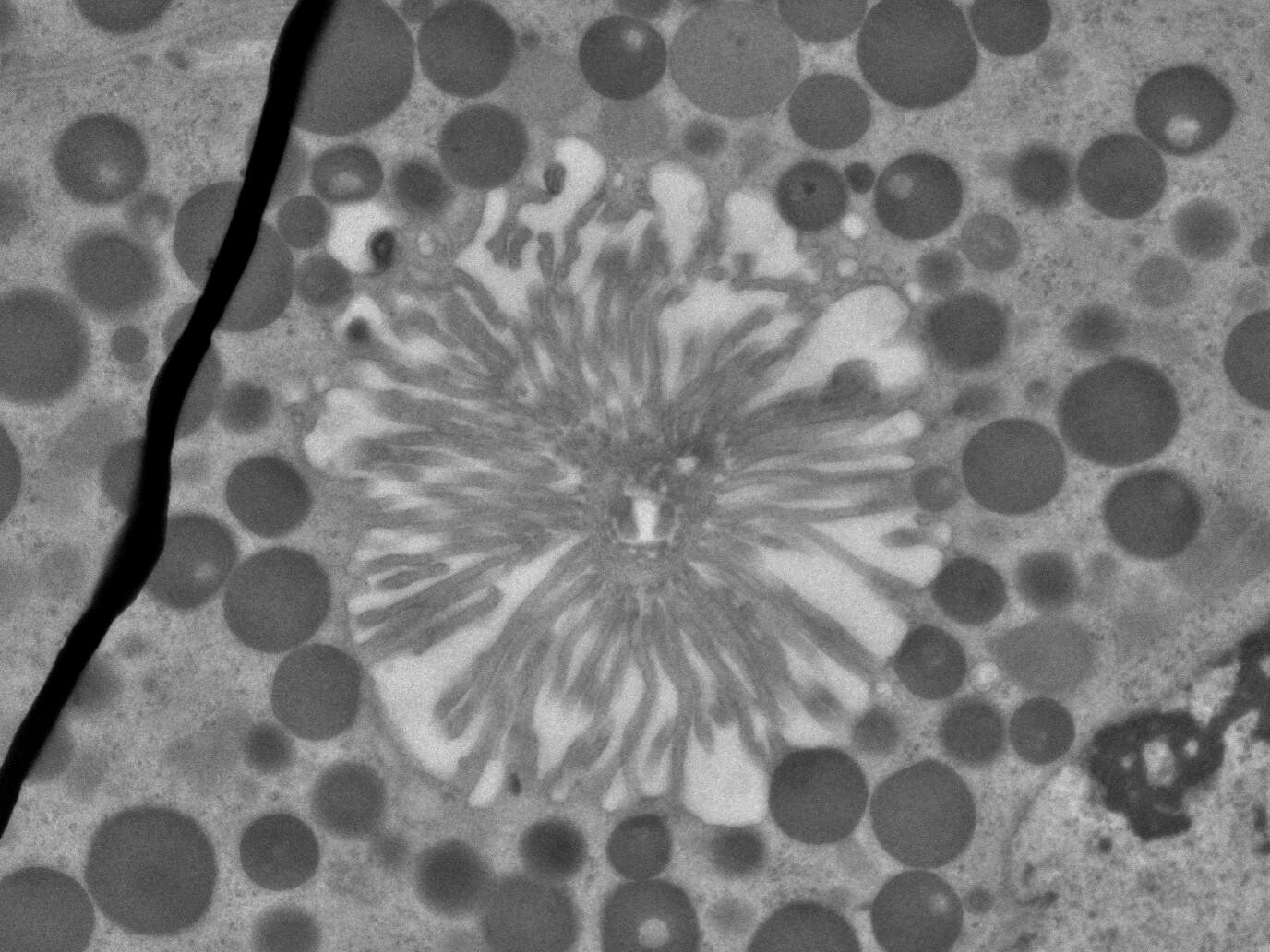This black and white image appears to be a microscopic view of cells or some kind of artistic design mimicking such structures. Dominating the center is a large, flower-like circular object, primarily white, with numerous lines radiating inward to a white core. Surrounding this central figure are numerous smaller circular shapes, mostly dark gray to black, which give the impression of cellular forms. A prominent black, diagonal line runs down and to the left of the image, adding a contrasting element. Additionally, the background features an assortment of tiny specks scattered throughout, particularly in the bottom left and lower right corners, providing a granite-like texture to the overall composition. The image contains no text or color aside from its grayscale hues.